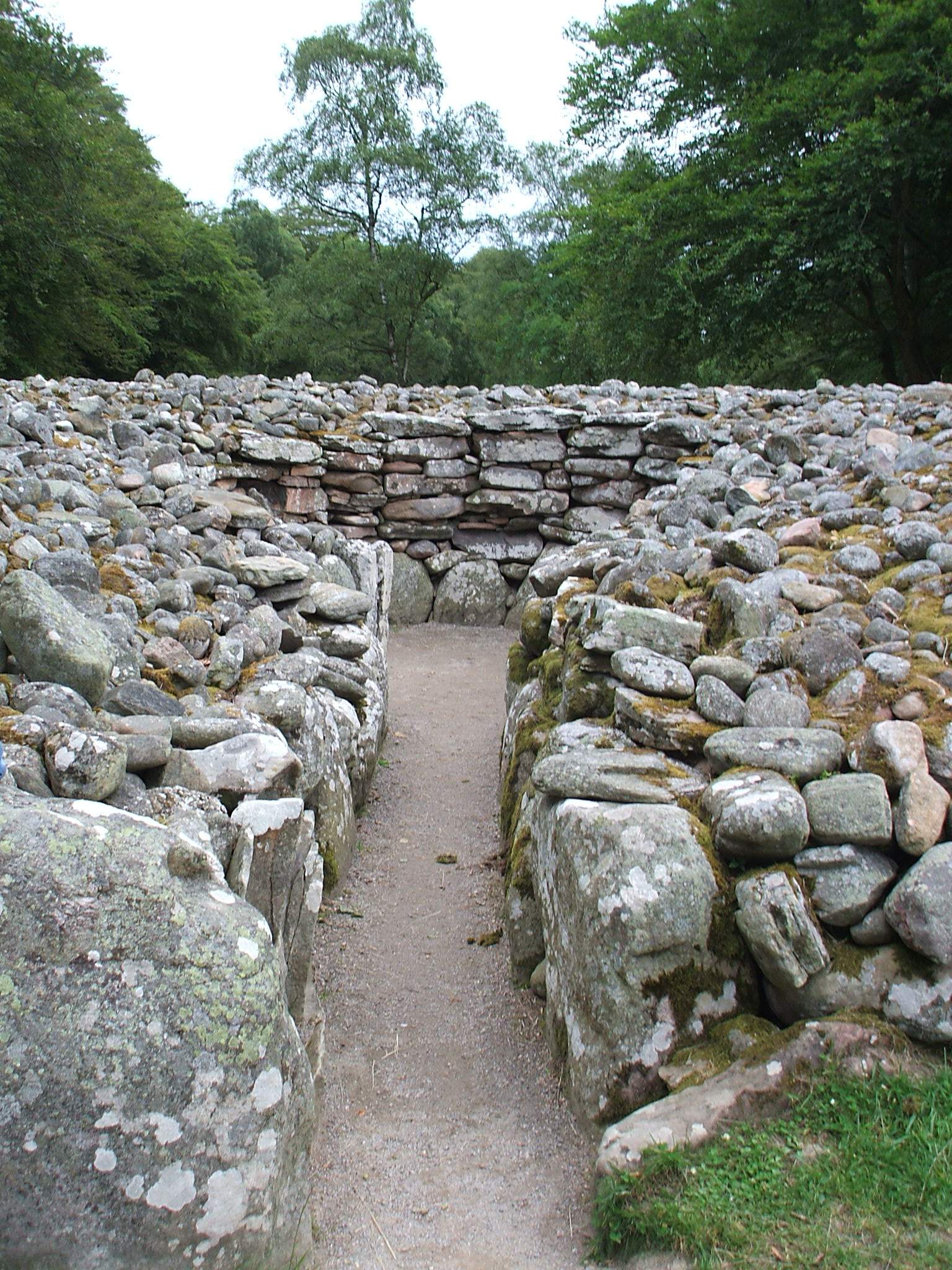The full-color photograph, taken outdoors in natural daylight, showcases a vertically rectangular scene with a clear and detailed view. The upper center of the image features a vibrant blue sky framed by lush green trees extending from the upper left and upper right. The focal point is an ancient, archaeologically significant stone structure situated midway down the photograph. 

This structure, constructed from meticulously stacked rocks, forms an open-air room with no roof, evocative of old city ruins from centuries past. Leading into this space is a narrow walkway flanked by walls of piled stones on either side. As the path proceeds, it encounters a horizontal barrier of rocks that forces a choice to go either left or right, adding a maze-like quality to the scene. These rock walls are adorned with patches of moss and sprigs of grass, highlighting the passage of time. Farther in the background, the green foliage of various trees can be seen against a white sky, suggesting a cloudy day. The entire composition combines natural and man-made elements, creating a vivid and historically rich tableau.